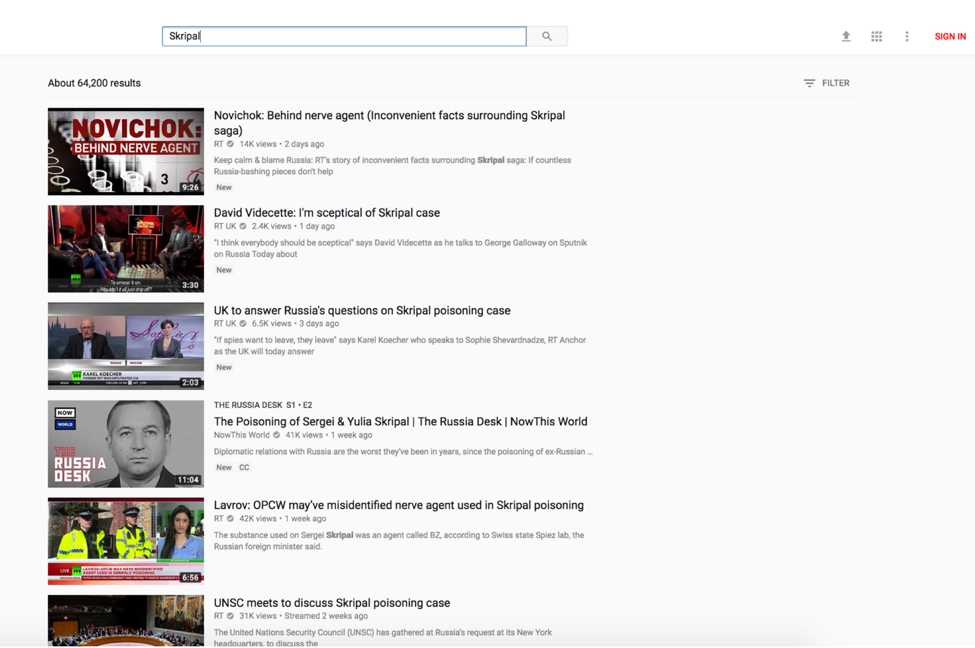This screenshot captures a page that mimics the layout of YouTube but isn't actually YouTube. At the top of the page, there is a distinct search bar, indicative of a search results page. Directly below the search bar, a line mentions "About 64,200 results." The search query has yielded six video results, each from different news channels. 

The first video in the list is titled "NevoChalk behind NerveAgent," published by RT News, which has a verified checkmark. This video has garnered 14,000 views and was uploaded 2 days ago, marked with a "New" tag. 

Next is a video from David Videsetti titled "I'm Skeptical of Scribble Case," published by RT UK. It has a much lower view count of 2.4 views and was uploaded just one day ago, also featuring the "New" tag. 

Skipping ahead to the last video in the list, it's titled "UNSC Meets to Discuss Scribble Poisoning Case," and was streamed two weeks ago by RT News. This video has accumulated 31,000 views. The description mentions that the United Nations Security Council convened at Russia's request at its New York headquarters to address the Scribble poisoning case.

To the right of the search bar at the top, there's an upward arrow icon and a grid icon, followed by a "Sign In" link. Beneath the "Sign In" link, a filter icon is visible. All this is presented on a predominantly white page background.